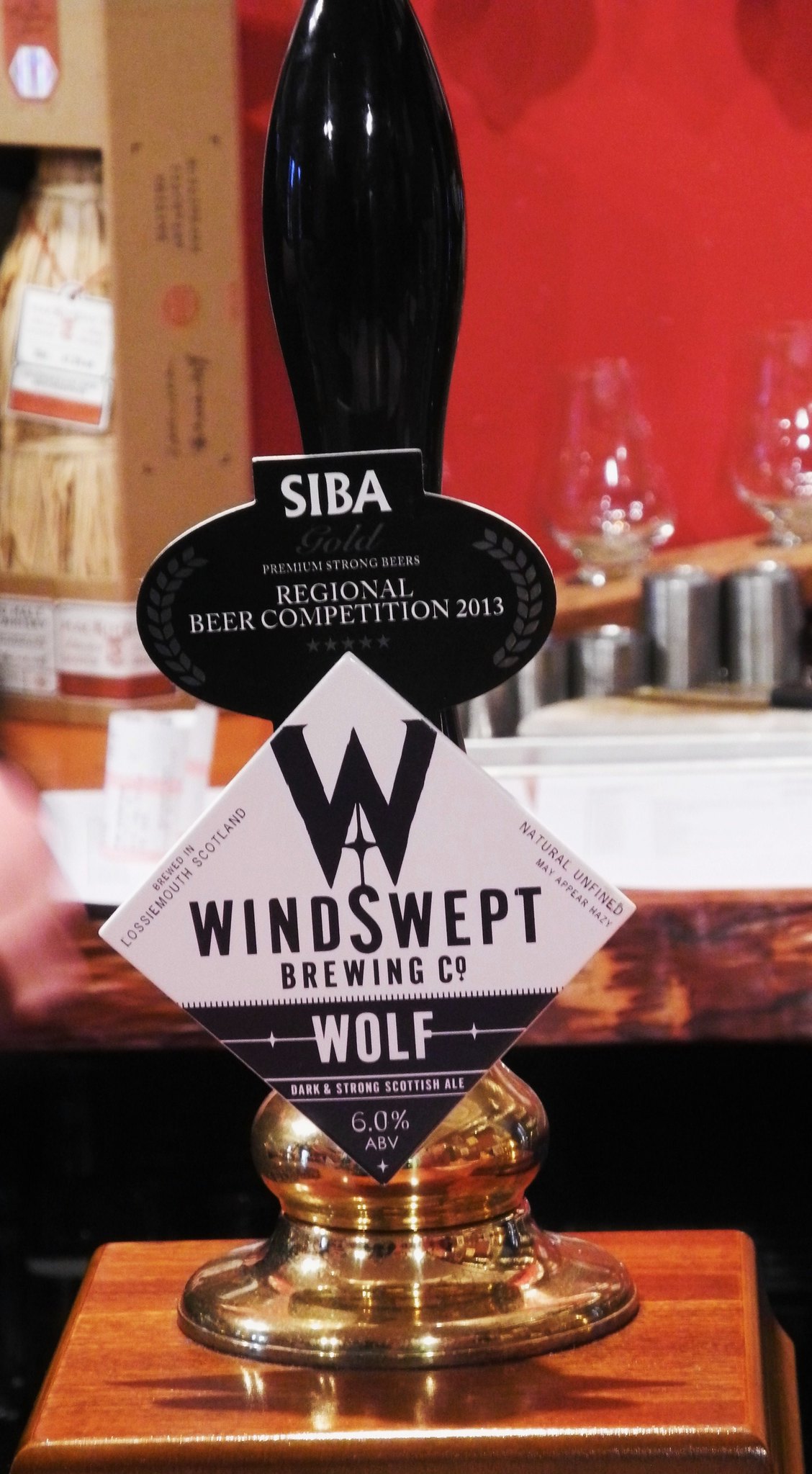The image depicts a detailed and meticulously crafted beer tap serving as an award on a wooden pedestal. The base is adorned with a lustrous gold finish, giving it an elegant and prestigious appearance. Atop the pedestal, the tap handle boasts a glossy black, tapered oval design, enhancing its sophisticated aesthetic. The centerpiece of the award features two prominent plaques. The diamond-shaped plaque proudly displays the "Windswept Brewing Co" logo and information, including "brewed in Lossiemouth, Scotland," "natural unfined, may appear hazy," and the beer’s specifics: "Wolf Dark and Strong Scottish Ale, 6% ABV." Above it, a smaller oval plaque reads "SEBA Regional Beer Competition 2023 Premium Strong Beers," indicating the recognition it received. The backdrop suggests a brewery setting with barware and packaging subtly blurred, contributing to the award’s contextual authenticity. This photograph captures the realism and artistry in the crafted award, celebrating the brewing excellence of Windswept Brewing Co.